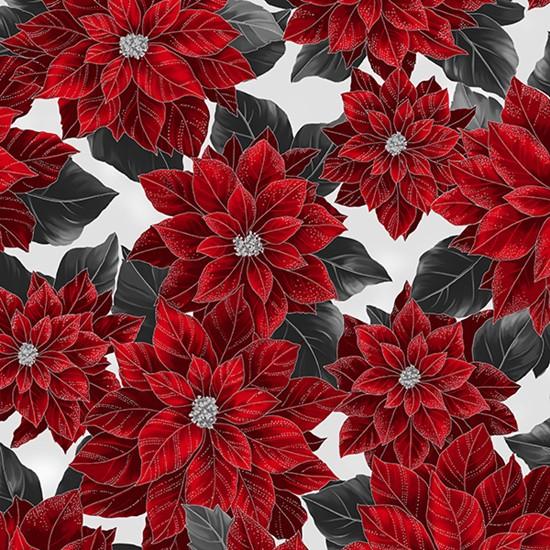The image depicts a detailed, hand-drawn illustration of poinsettias on what appears to be Christmas wrapping paper. The design features a white background crowded with large and medium-sized poinsettias, approximately 10 in total. The poinsettias are rendered with vibrant, dark red bracts, which are often mistaken for petals, and almost black, dark green leaves that lend a somber, yet elegant touch to the overall composition. The centers of the flowers contain distinguishing white specks. While most flowers are in full bloom and prominently displayed, some are partially cut off at the edges of the square image, creating a sense of an abundant and random arrangement rather than a repetitive pattern. The dark colors of the leaves and bracts contrast strikingly with the plain white background, ostensibly achieving a style that is sophisticated rather than traditionally bright and cheerful for Christmas themes.